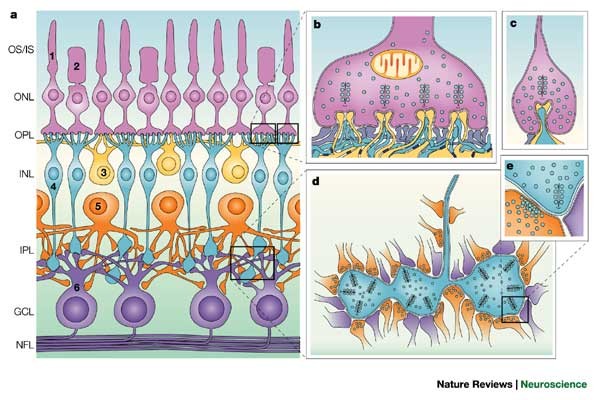The image is a detailed scientific diagram related to neuroscience, labeled with "Nature Reviews Neuroscience" at the bottom. It demonstrates a series of processes or structures, divided into five sections labeled A, B, C, D, and E. The color scheme includes purple, light blue, orange, and yellow.

Section A displays a column of labels on the left side: OSIS, ONL, OPL, INL, IPL, GCL, and NFL. The diagram is multicolored with the bottom section lined in purple showing purple circular structures interconnected with tendril-like shapes. Above these, blue, purple, and yellow teardrop shapes are also interconnected by tendrils.

Section B shows a purplish, tooth-like shape with intertwined blue and yellow lines, alongside a gold-colored circular section with gold lines inside.

Section C continues this theme, presenting a smaller teardrop-shaped purple image with blue and yellow lines running through it and white specks scattered across.

Sections D and E depict blue cellular structures, seemingly amoebic in nature, with purple and orange tendrils pressing against their edges. 

The diagram appears to provide an educational visual breakdown of a complex neuroscientific process, possibly related to brain or eye structures, as conjectured from the colors and labeled sections.